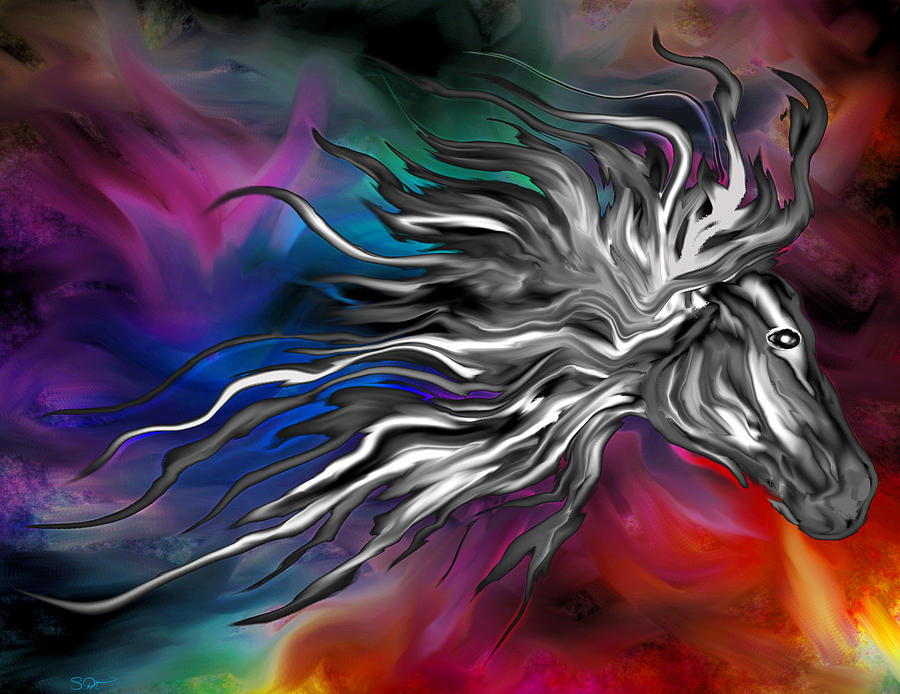In this vibrant, wide vertical artwork, likely a computer-generated digital piece, swirling colors blend seamlessly across the background, creating a striking visual palette. From the top left down to the center, rich shades of purple, blue, and teal intermingle with hints of dark gray, while the bottom right half bursts with dark oranges, reds, and dark yellows, flecked with touches of green and purple. The diagonal interplay of these rainbow hues makes the background a mesmerizing mixture of warm and cool tones.

Dominating the center of the image is a meticulously crafted horse's head, depicted in contrasting black and white or dark and light gray shades. The horse's head is angled slightly downward, with its snout directed towards the lower right corner. Its eye, stark and expressive, adds a focal point of intensity. The horse’s mane flows wildly, extending in dynamic streams that reach towards every corner of the canvas, suggesting motion and energy. This ethereal, floating creature-like form stands out against the colorful chaos, grounding the otherwise abstract composition in a recognizable figure.